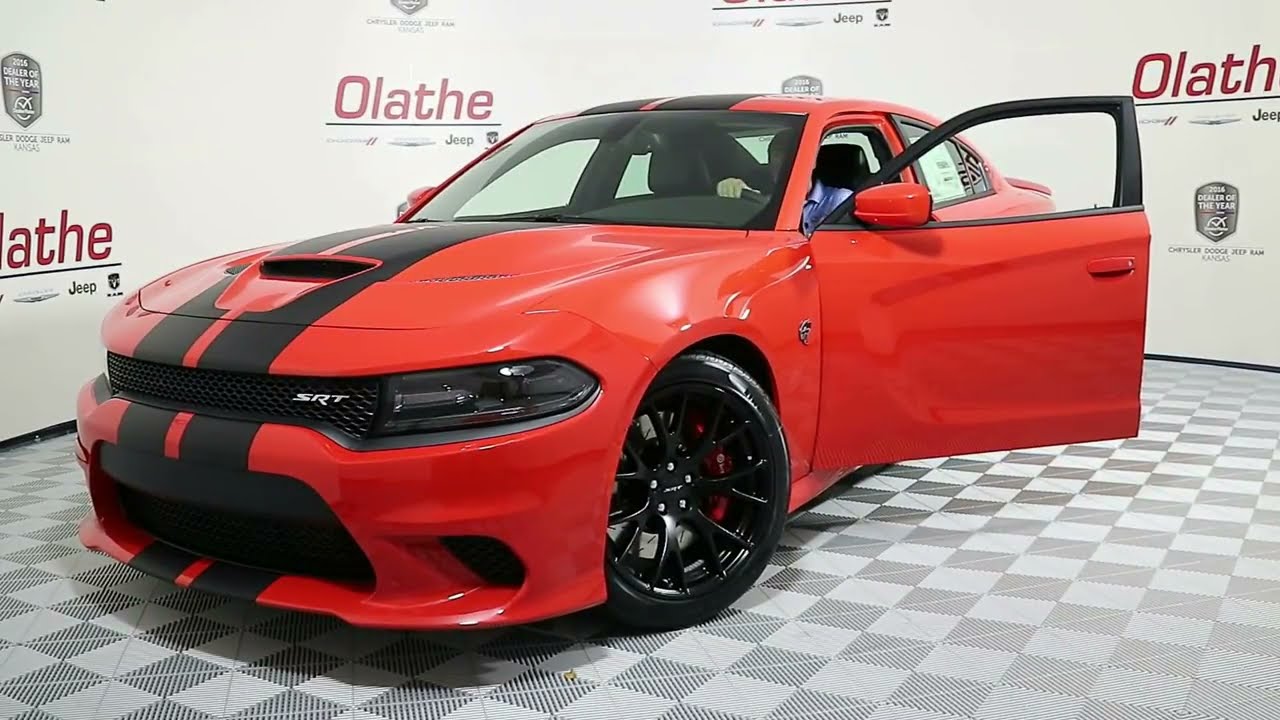The image depicts a Dodge SRT muscle car showcased indoors, likely at a car show. The car, painted in a very dark shade of orange with a double-sided black stripe running down its center, occupies the middle of the image at a diagonal angle, revealing both its front and side. It is parked on a multi-textured, checkerboard-tiled floor composed of black and white squares. The car features black rims, and a driver wearing a light blue dress shirt is seated in the driver’s seat with the door open.

In the background, an advertisement-laden wall is visible, featuring various promotional graphics including the notable word "Olathe," which could refer to Olathe, Kansas, or the name of the company hosting the show. Other advertisements mention “Jeep” and “Dealer of the Year,” although the specific year remains unreadable. The overall setting and the specific details of the backdrop suggest this is an indoor car show dedicated to showcasing this impressive vehicle. The visible color palette from the ad banners includes red, black, gray, maroon, and silver.